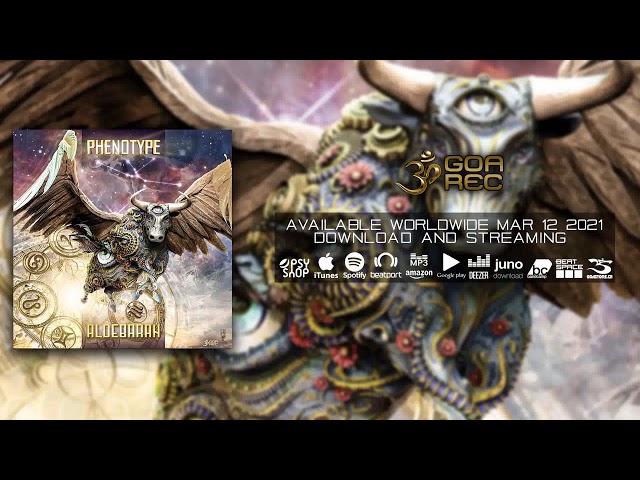This digital artwork serves as an intriguing album cover for "Phenotype," prominently featuring a fantastical bull with large wings and intricate armor adorned with gold and blue hues interspersed with pink flowers. The bull's defining feature is a single large eyeball in the center of its forehead, lending an otherworldly vibe to the image. Positioned towards the front, the bull appears to be floating midair with its wings spread, gazing slightly to the right.

The album cover presents a mixture of vibrant colors, including brown, turquoise, purple, tan, gray, gold, red, white, green, and light shades, creating a visually captivating scene. The layout includes a magnified version of the cover taking up most of the space, with a smaller duplicate image placed in the left middle section of the frame.

Text on the cover informs viewers that the album "Phenotype" will be available worldwide on March 12, 2021. It can be downloaded or streamed on various platforms, including iTunes, Spotify, Amazon, Google Play, Steam, Beatsplit, Juno, BC, Squeeze, and more, under the label "GOAREC."